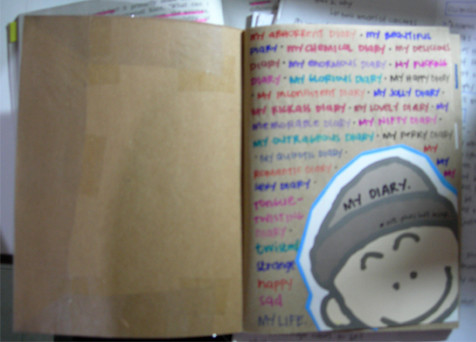The image shows a low-resolution photograph of an open journal, appearing to be a work in progress. The left-hand page resembles brown cardboard or paper bag material adorned with pieces of clear tape but remains otherwise unused. The right-hand page is densely packed with multicolored statements, written in an array of markers including red, blue, orange, teal, brown, and black. Although the exact text is indiscernible due to the image's resolution, the format consists of various short phrases each rendered in a different color. Dominating the bottom right corner of this page is a whimsical illustration, possibly a sticker, featuring a simple character with a white face, tiny beady eyes, raised eyebrows, and a single-line smile. The character dons a black beanie cap with the words "My Diary" inscribed prominently in black marker. The entire scene hints at a creative and personalized journaling process.